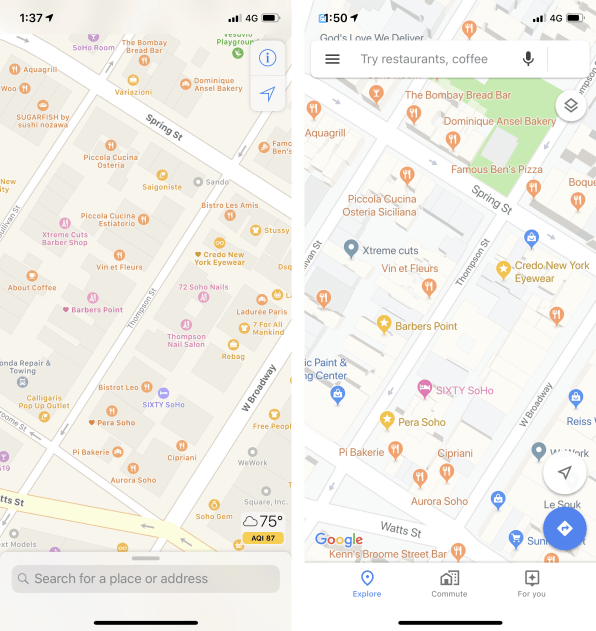The image showcases two screenshots of a smartphone displaying a map application, evident from the visible status bars at the top that show the time, battery level, Wi-Fi strength, and 4G connection. The left screenshot, timestamped at 1:37, features a map with a search bar at the bottom reading "Search for a place or address." Various locations are marked on the map, including Vin et Fleurs, Piscola, Coquina, Osteria, Sando, Bistro Les Amis, 72 Soho Nails, Thompson Nail Salon, and 60 Soho. The areas on the map have a beige tint, and the temperature in the lower right corner reads 75 degrees.

The right screenshot, timestamped at 1:50, also displays a map of presumably the same area but with a different visual style. The background appears whiter compared to the left image's beige filter. The map highlights different locales such as Barber's Point and 60 Soho, using a distinct style and font. A search bar located at the top prompts users to "Try restaurants and coffee," and includes a microphone icon for voice input. Additional interface elements include a white compass button and a blue direction button. At the bottom of the screen, navigation options such as Explore, Commute, and For You are visible.